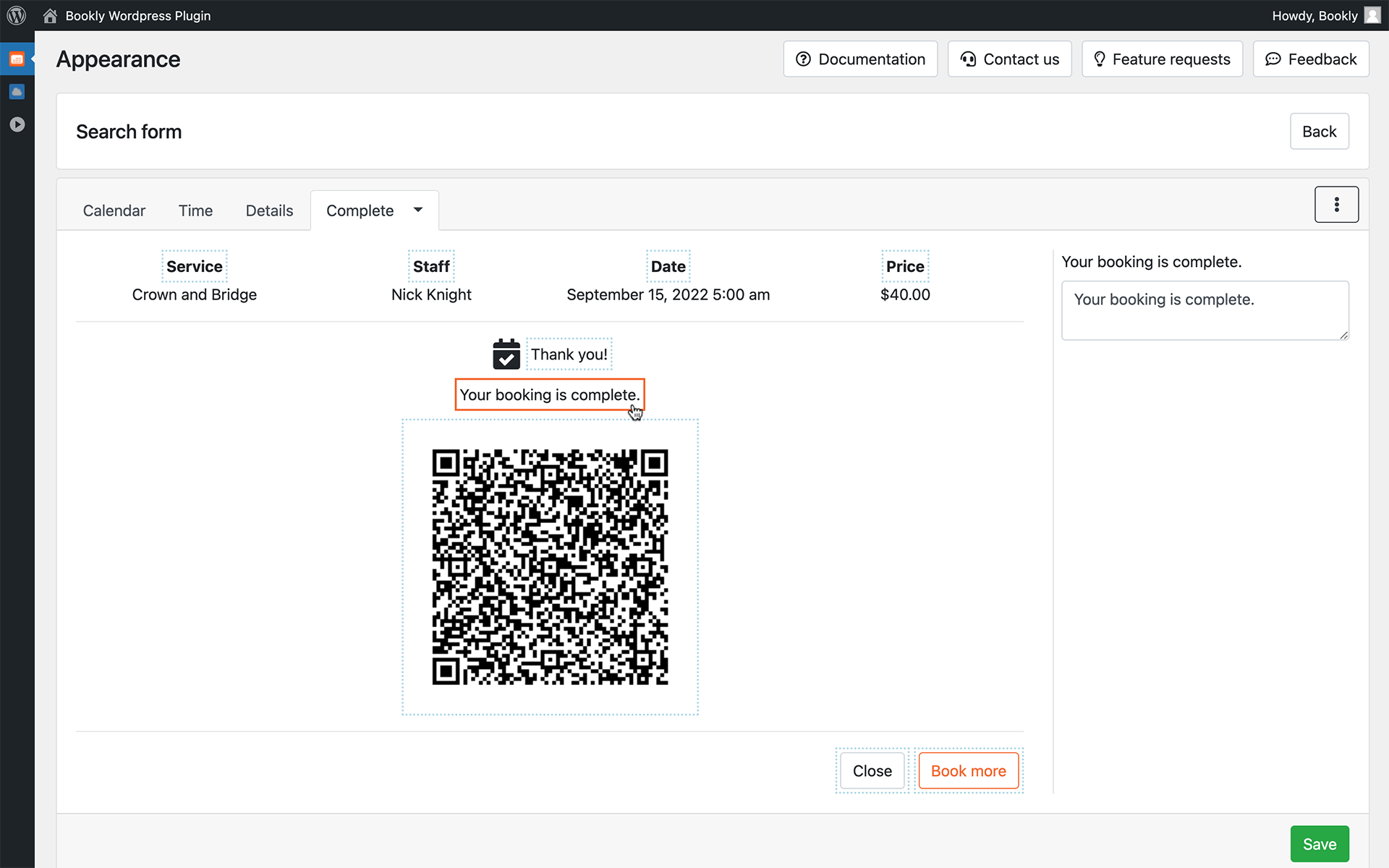Screenshot of a WordPress Website Interface

At the top of the screen is a horizontal black bar, featuring a gray circle with the WordPress icon situated on the left side. To the right of the icon is a gray house icon, followed by the text "Bookly WordPress plug-in" on the right-hand side. On the far right of the black bar, the text "Howdy Bookly" appears in white, adjacent to a gray profile square.

The main background of the page has an off-white or light gray hue. Prominently, there are multiple white sections with inserted black text. In the top-left corner, bold black text reads "Appearance."

In the upper right corner, three horizontal white bars are visible with labels in black text: "Documentation," "Contact Us," "Feature Request," and "Feedback."

Beneath this, there is a white text box area with "Search Form" written in black on the left side. To the right is a white button with "Back" written in black.

Further down, on the left side, there are three labels: "Calendar," "Time," "Details," and "Complete," each accompanied by a downward arrow. The "Complete" label is selected, and underneath it, on a white background, several details are listed from left to right:
- Service: Crown and Bridge
- Staff: Nick Knight
- Date: September 15, 2022, at 5 a.m.
- Price: $40

To the right of these details, it states "Your booking is complete."

Beneath this section, there is a prominently displayed QR code outlined in red, accompanied by the message "Your booking is complete, thank you."

In the bottom right corner, buttons are visible: a white "Close" button with black text on the left and a white "Book More" button outlined in red with red text on the right.

Additionally, the black bar extends down the left side of the screen, showing a series of three icons from top to bottom: an orange icon, a blue icon, and a white play button icon.